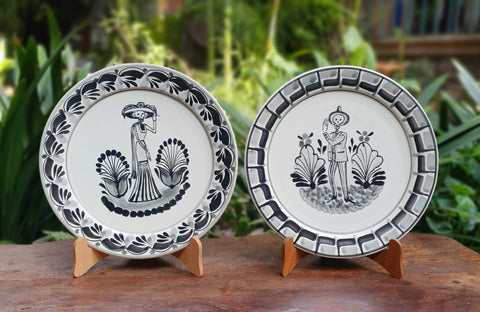The image features two ornate plates displayed on wooden stands atop a brown marble surface with a marbled pattern in various shades of brown, including light, dark, and pinkish tones. In the background, lush greenery and broadleaf plants can be seen, possibly alongside a building. The left plate features intricate blue and white floral designs around its edge, with a central depiction reminiscent of the Day of the Dead: a skeleton woman wearing a large hat and a long dress, flanked by flowers and beads. The right plate showcases a skeleton man in a suit, with plants on either side and a border pattern that resembles shells. The wooden stands holding the plates add a tasteful touch, complementing the earthy tones of the marble surface.